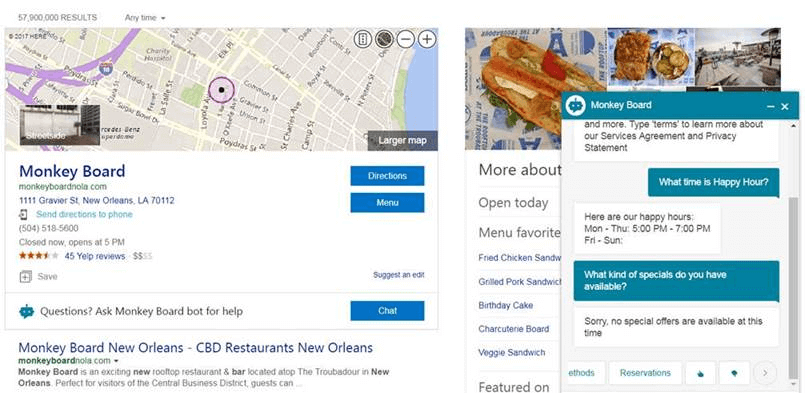The image is a horizontally rectangular screenshot of a Google search page. On the left side of the image, a box displays a map at the top, with "Monkey Board" indicated beneath it as a location situated in New Orleans. On the right side of the box, there are clickable options for "Directions," "Menu," and "Chat." The chat window is open, occupying the right side of the frame.

In the chat window, a customer inquires about the establishment's happy hour. Monkey Board replies with the following information: “Here are our happy hours. Monday through Thursday, 5 to 7 PM. Friday to Sunday, there are no times listed.” The conversation continues with the customer asking about special offers, to which Monkey Board responds, “Sorry, no special offers are available at this time”.

Below the chat, there are buttons for making reservations and providing feedback, indicated by thumbs up and thumbs down icons.